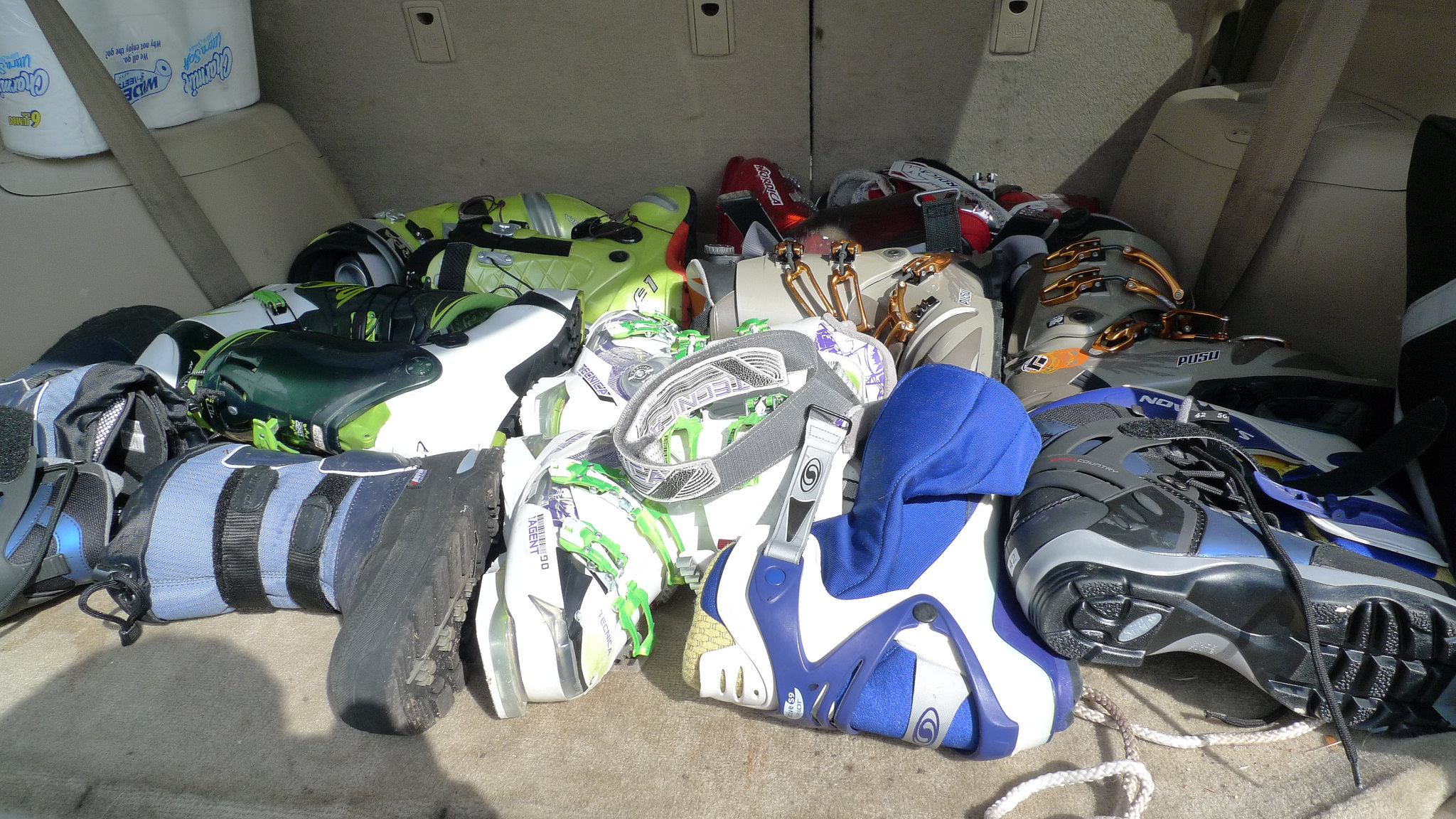The photograph depicts the cluttered interior of a car trunk, showcasing a collection of colorful ski boots strewn haphazardly across a dirty gray, carpeted surface. The boots, appearing in a range of colors including white, blue, purple, green, red, gold, orange, black, and brown, are chaotically piled on the seat and trunk floor without any visible patterns or organization, rather than neatly arranged. Additionally, a package of white toilet paper with blue writing on the clear plastic wrapping can be seen positioned on a surface where the wheel well rises. Seat belts are visible in the top left and right corners of the image, reinforcing the setting as the interior of a vehicle.